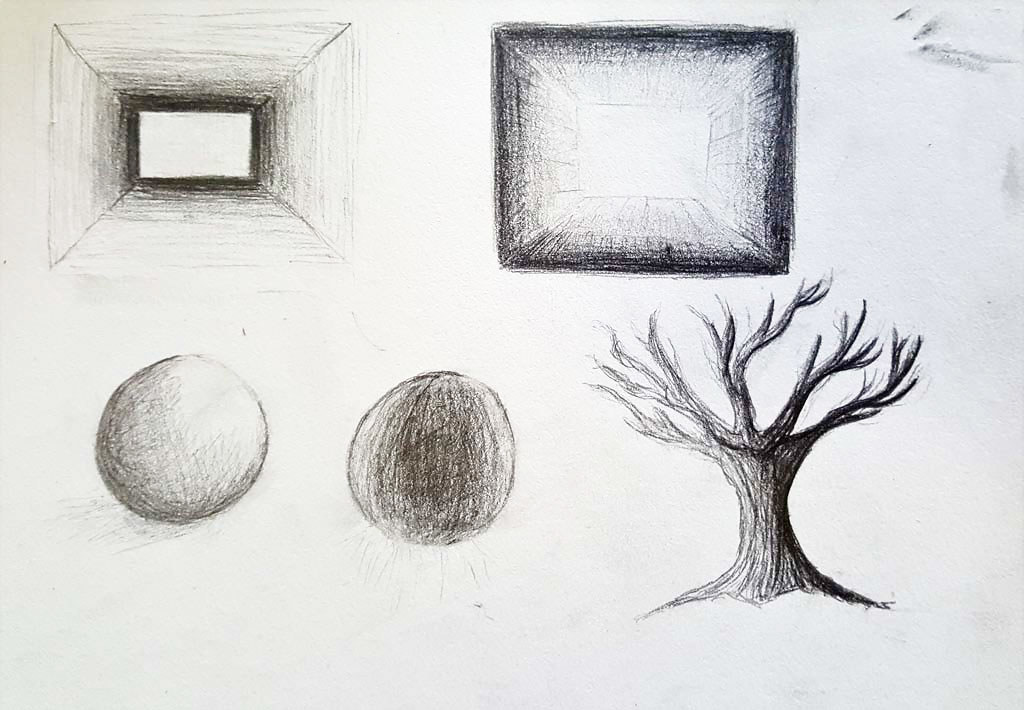The image depicts a detailed charcoal and pencil sketch composition on plain white paper, enhanced with subtle colored pencil or crayon accents. Prominently in the bottom right corner, a small tree trunk with barren branches is depicted, shaded to suggest a light source. To the left, two spheres are presented: one is partially shaded on the left side, and the other is completely filled in black. In the upper left corner, a large square recedes into a smaller square, creating the illusion of a hallway with a bright white patch at the distant end. The upper right side features another square, shaded along the edges, encasing a smaller square which appears to emit light from its center.